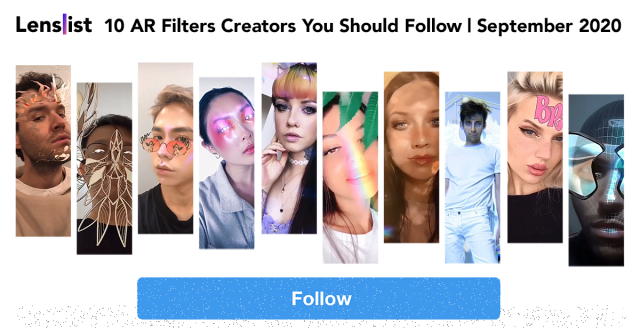This landscape-oriented promotional image appears to be an ad for a social media channel called "Lens List." At the top of the image, there's black text that reads "Lens List" and "10 AR filter creators you should follow September 2020," indicating that the content is from September 2020. Central to the image is a row of portrait photographs displaying a diverse group of young influencers using various augmented reality filters. Notable details include a man with dark hair covered in leaves, another man with a bird on his face, an Asian man with flaming red glasses, and an Asian woman adorned with pink and purple makeup. Additionally, there is a Caucasian girl with colorful bangs, a Latino girl with a white blur on her face, a Caucasian girl with long brown hair and gray eyes, a Hispanic man dressed entirely in white, another Caucasian girl with blonde hair and a caption on her forehead, and an African American man with a grid overlay. Below these photographs, a prominent blue button with the word "Follow" in white lettering suggests an invitation for viewers to engage with the featured AR creators on social media.